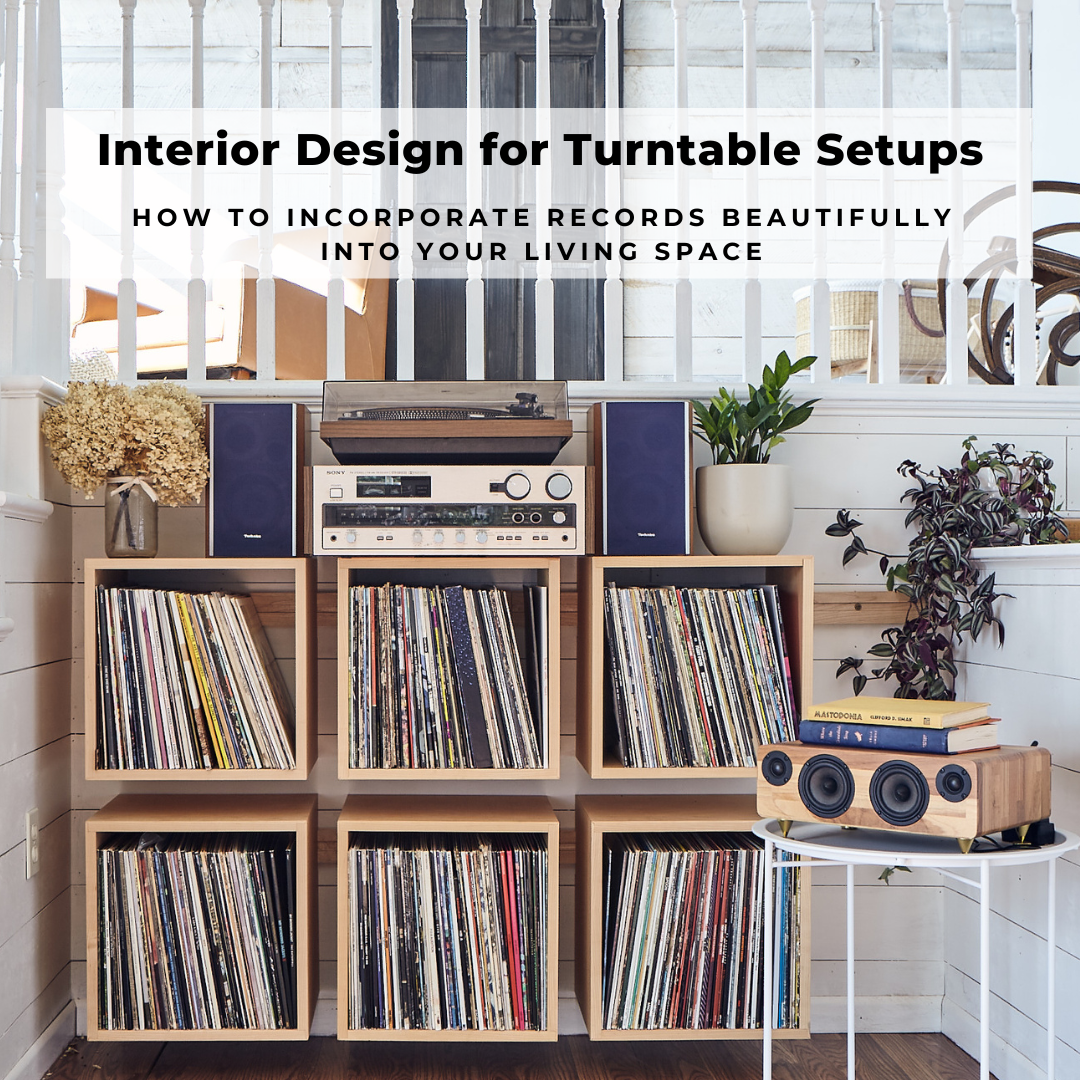The cover image showcases an interior design catalog titled "Interior Design for Turntable Setups: How to Incorporate Records Beautifully into Your Living Space," with these words elegantly written in bold black font. The setting features a sophisticated arrangement perfect for audiophiles and design enthusiasts alike. Central to the scene are six large wooden shelves filled with an array of record albums. Atop these shelves sits a silver stereo system paired with a vintage brown turntable. Flanking this setup are two rectangular speakers with blue faces. The aesthetic is augmented by greenery, featuring a potted plant and a set of dried flowers on either side. Additional elements include a dangling plant in one corner and a sleek, white background with white banister handles visible above. The scene is further enriched by the presence of a subwoofer to the bottom right, which rests on a light brown box, accompanied by two books. This meticulous setup exudes a sense of harmony and balance, artfully merging music and interior design.